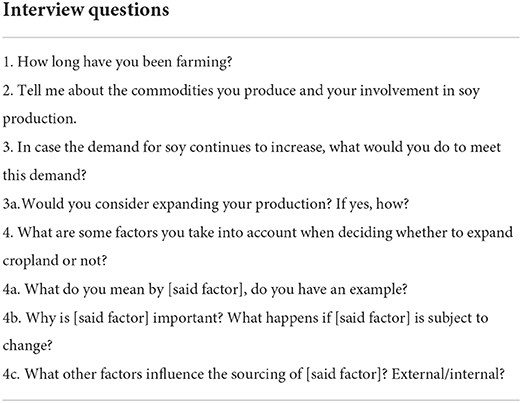This image depicts a detailed list of interview questions, each meticulously organized and presented under the header "Interview Questions" that is prominently printed in bold black text at the top of the page. A faint gray line separates this heading from the actual questions, providing a structured layout.

The questions are enumerated as follows:

1. **How long have you been farming?**
   
2. **Tell me about the commodities you produce and your involvement in soy production.**
   
3. **In case the demand for soy continues to increase, what would you do to meet this demand?**

   3A. Would you consider expanding your production? If yes, how?

4. **What are some factors you take into account when deciding whether to expand cropland or not?**

   4A. What do you mean by said factor? Do you have an example?
   
   4B. Why is said factor important? What happens if said factor is subject to change?
   
   4C. What other factors influence the sourcing of said factor (external, internal)?

The structure reveals that questions 4, 4A, 4B, and 4C are extensions of the broader query regarding factors influencing the expansion of cropland, making the list appear more comprehensive than a simplistic four-question format might suggest.